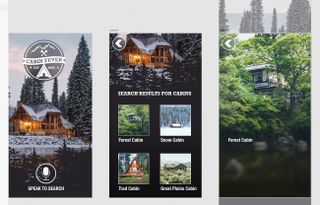The image contains several visual elements and overlays, each contributing to a detailed composition:

1. **Background**: The top three-fourths of the image features a solid gray background, extending to the right side.

2. **Overlays**: Positioned on top of the gray background are three distinct pop-up images or scans resembling pages from an old brochure.

3. **First Pop-up (Leftmost)**:
   - **Scene**: Depicts an enchanting, lightly dusted snow-covered log cabin with a tan roof. Massive evergreen trees dominate the background.
   - **Logo**: A green circular logo is centered at the top, containing the text "Cabin Fever" (though slightly difficult to discern) surrounding a white circle with a green text.
   - **Additional Element**: At the bottom, there is a white circle featuring a desk microphone icon and the text "Speak to Search."

4. **Second Pop-up (Center)**:
   - **Scene**: Displays the same cabin, but this time zoomed in from a slightly different angle, making the evergreen trees appear larger at the bottom.
   - **Text**: Beneath the image, white text reads "Search Something for Cabins." Below that, there are four small pictures showcasing various cabins.

5. **Third Pop-up (Rightmost)**:
   - **Scene**: A grayscale image featuring an elegant treehouse surrounded by more tropical-looking trees, positioned under more gray-toned trees.

This composition blends a serene, rustic aesthetic with modern interactive elements, evoking a nostalgic yet functional feel.